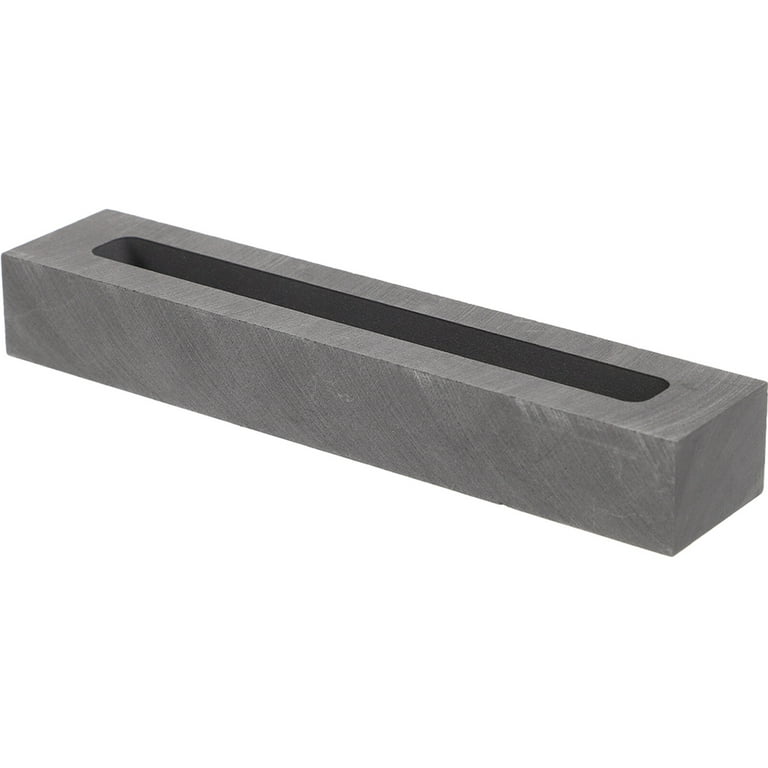The image displays a gray, elongated rectangular brick or block positioned against a solid white background. The block, which has the appearance of being crafted from stone, features a prominent, dark rectangular hole running along its length, suggesting considerable depth, though it is unclear if this hole passes entirely through the block. The texture of the stone shows a marbling effect with swirling lines that imply it may have been cut by a saw. The object is oriented at an angle, stretching diagonally from the top left to the bottom right of the image. The overall scene is simple, with no additional writings or objects present in the picture, highlighting the solitary and somewhat ambiguous nature of the block.